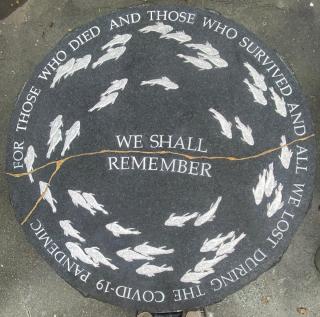The image depicts a commemorative gray stone circle mounted on a concrete background. Inscribed in white text, the central message reads, "For those who died and those who survived and all we lost during the COVID-19 pandemic, we shall remember." Surrounding the perimeter of the circle are white fish, creating a symbolic ring around the text. A prominent gold line runs horizontally across the middle of the circle, resembling a branch or crack. The setting and design appear to honor and remember individuals affected by the COVID-19 pandemic, evoking both loss and resilience through its symbolic elements and somber aesthetic. The hues of slate, gray, white, and yellowish gold add to the poignant atmosphere of the memorial.